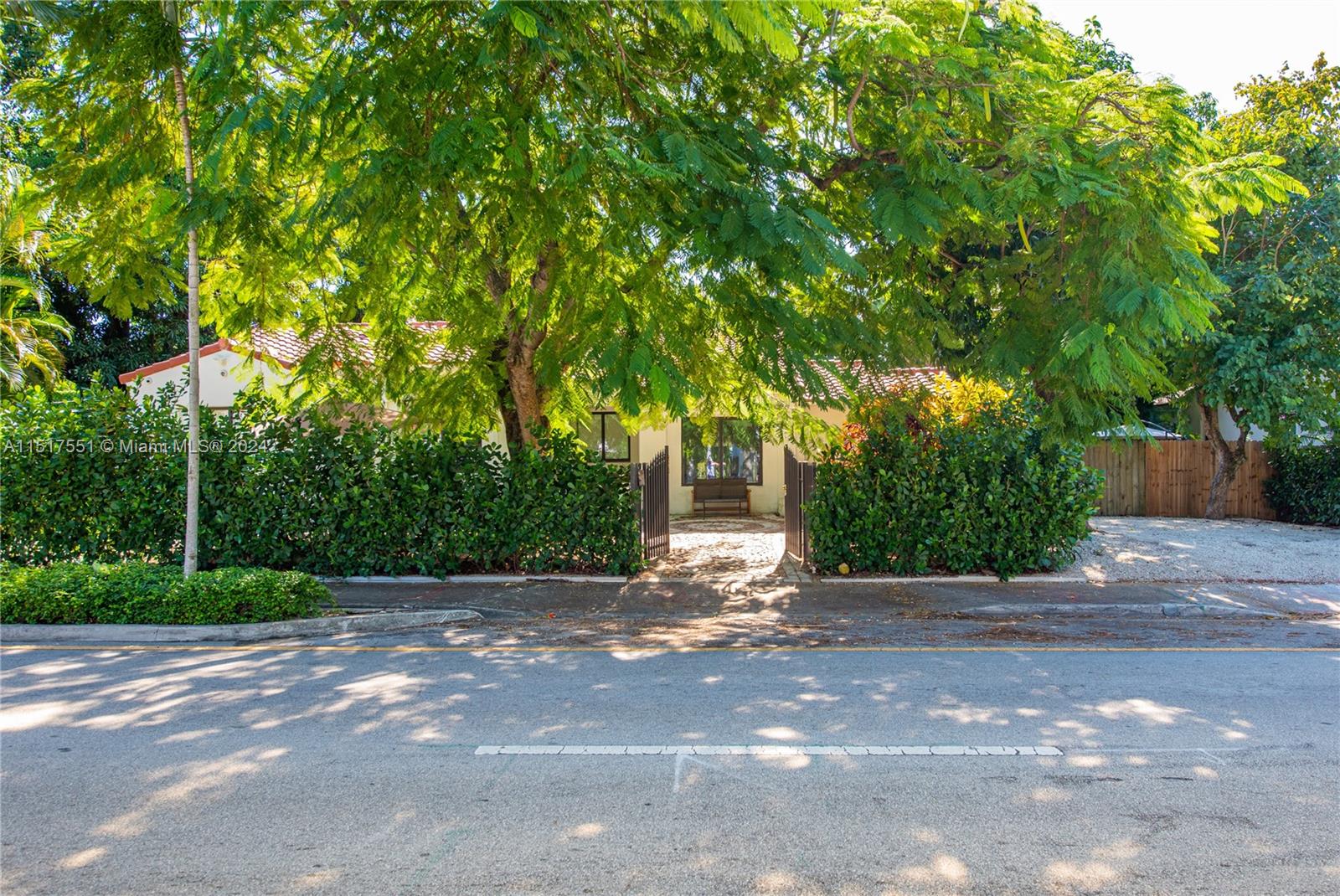This photograph captures a home viewed from the street, where the road is marked by a small median and remains empty. The house, which appears to be a light yellow or beige color, is partly obscured by a high fence and lush, tall green shrubs providing privacy. An open gate in the fence offers a glimpse of the front of the house, revealing a bench positioned in front of a main window. A large, overhanging tree sits prominently in the center of the yard, its broad canopy providing significant shade. To the right of the house, an empty driveway leads towards a brown wooden fence. The street itself is a mix of light and dark gray hues, and the bright sun indicates it is daytime. A watermark on the left side of the image reads "A-11-151-7551, Miami, MLS, 2024," hinting at the photo's origin. The image suggests the home needs some cleaning and maintenance.